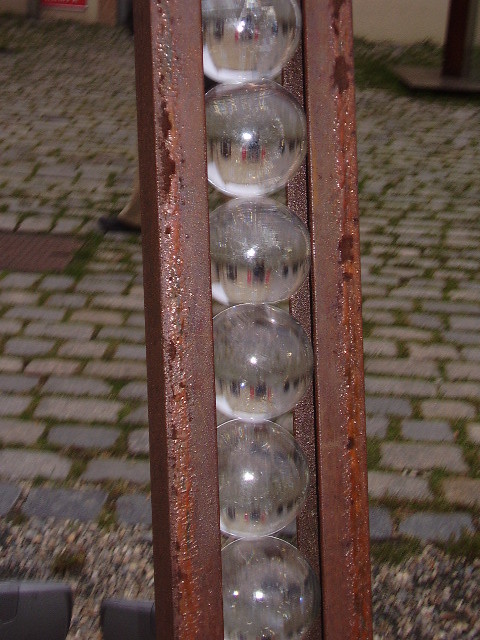The image displays an artistic water fountain that features a series of clear, circular glass or acrylic balls. These transparent balls are stacked and mounted within a metal channel, held upright by rusted steel or bronze poles on either side. The rust on the metal suggests prolonged exposure to water, enhancing its aged appearance. Water appears to trickle down the balls in a dribble effect, cascading into the base of the fountain. The background shows a weathered brick walkway with moss growing in the grout lines, indicating the outdoor setting. A passerby's black shoe and foot are partially visible behind the display, along with gravel at the fountain's base. The overall scene captures the blend of natural decay and artistic design, framed against a backdrop of light to dark gray pavement bricks and a wall with cream and hints of red coloration.